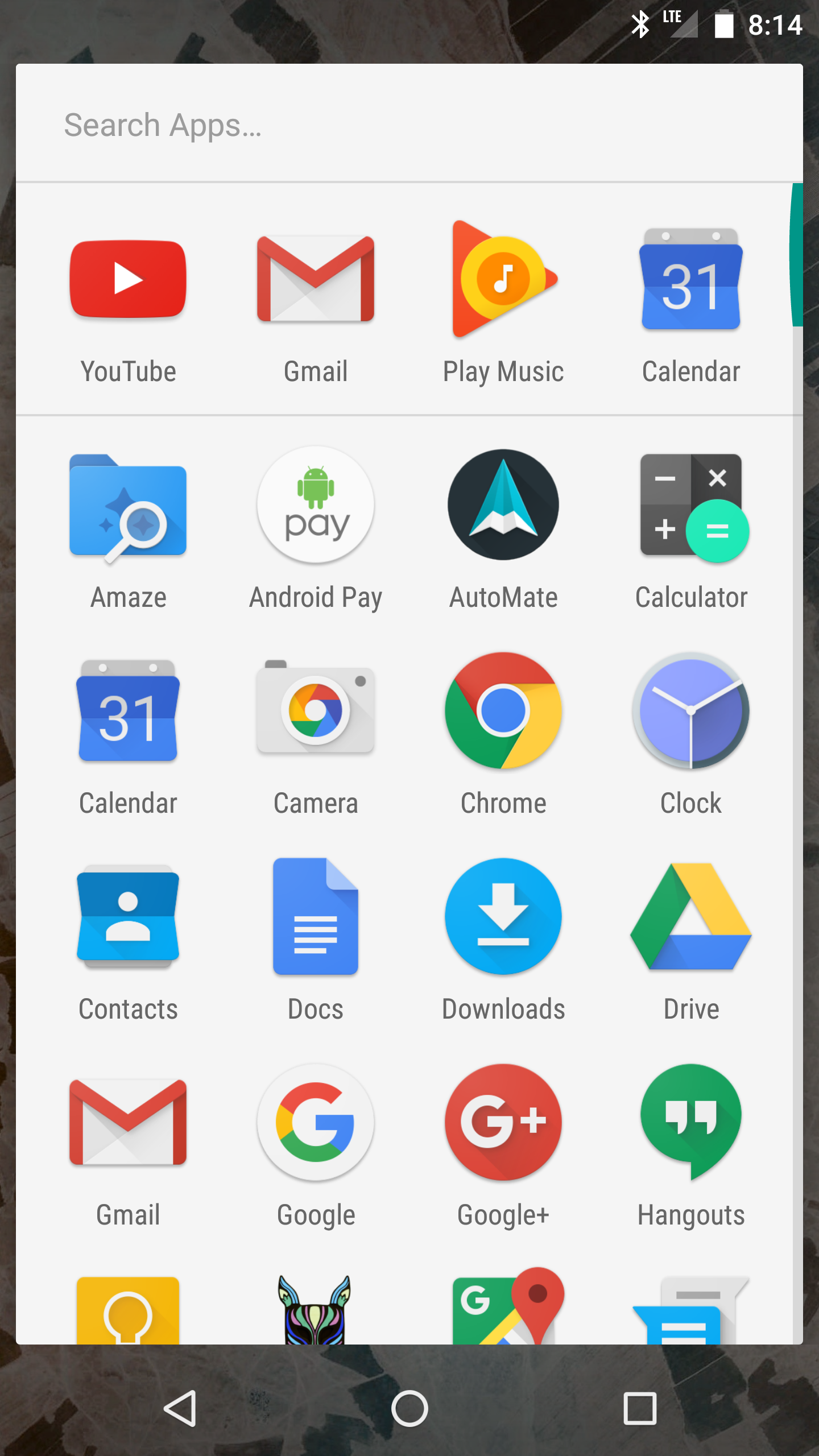The screenshot captures the home screen of someone's black smartphone, showcasing a variety of apps organized both by recent and alphabetical order. The screen has a white background in the app search area, delineated by gray lines separating different sections. 

Recent apps:
1. YouTube
2. Gmail
3. Play Music
4. Calendar

Following the gray line, the alphabetical list of apps includes:
1. Amaze
2. Android Pay
3. AutoMate
4. Calculator
5. Calendar
6. Camera
7. Chrome
8. Clock
9. Contacts
10. Docs
11. Downloads
12. Drive
13. Gmail
14. Google
15. Google+
16. Hangouts
17. Keep (Google Keep)
18. An app with an icon depicting a stylized face in yellow, green, red, and blue colors
19. Google Maps
20. An app with an icon featuring a blue page over a white page (likely Google Docs)

At the bottom of the screen, the navigation buttons include the back arrow, home circle, and recent apps square, all outlined in white.